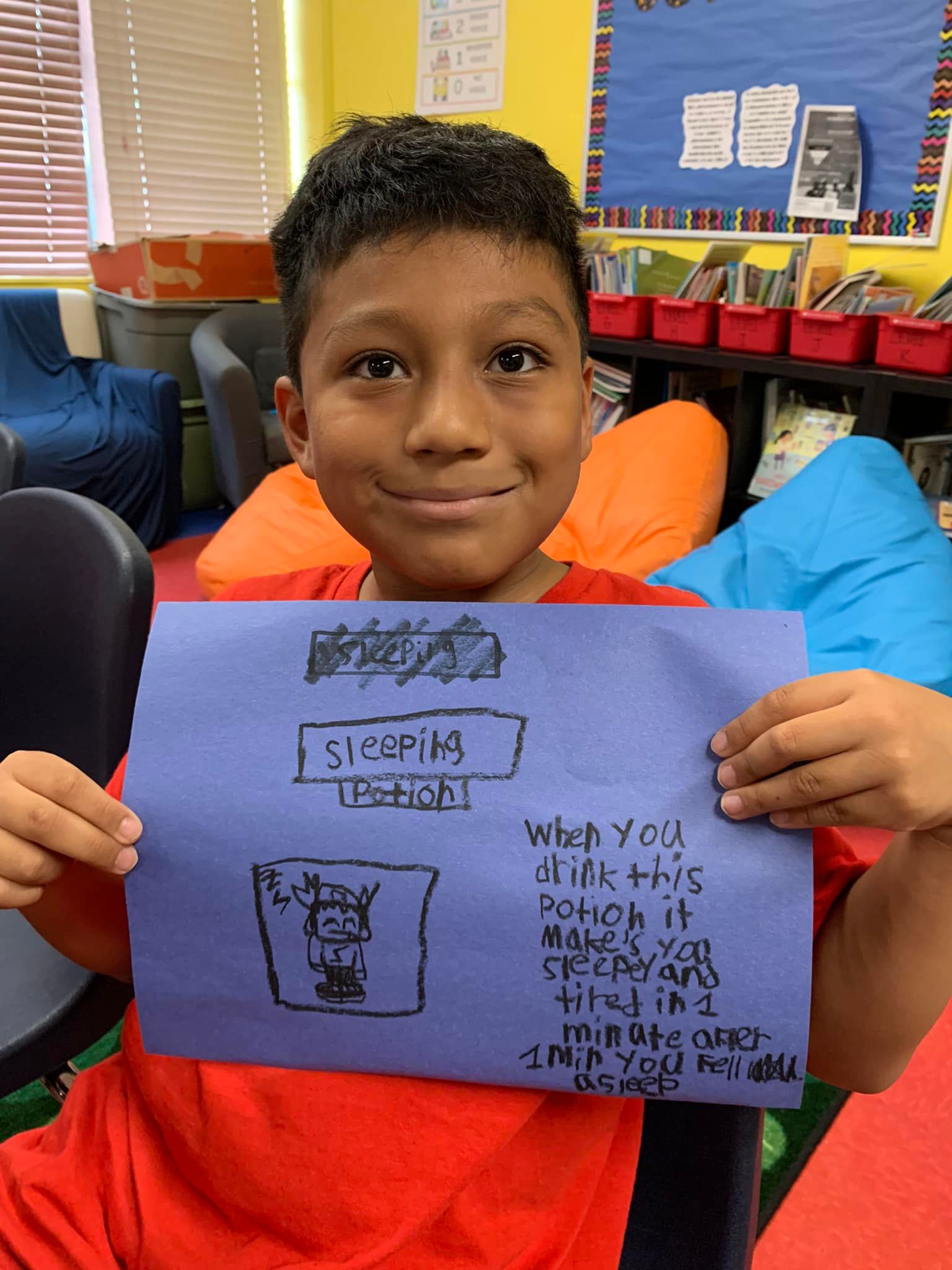The photograph captures a young elementary-aged boy at school, proudly displaying his artwork. He has short brown hair and is wearing a red t-shirt, smiling with his mouth closed. The piece of construction paper he holds is blue and features a creative drawing titled "Sleeping Potion." Initially, he wrote "sleeping," then crossed it out and rewrote it correctly. The artwork includes a black crayon drawing of a cartoon figure, presumably the boy, lying in bed. The accompanying text reads, "When you drink this potion it makes you sleepy and tired. In one minute after one minute you fell asleep," despite a few spelling errors. In the background, the classroom setting includes yellow walls, windows with shades, bean bags, a bulletin board with announcements, cubbies, and several books organized in plastic tubs.